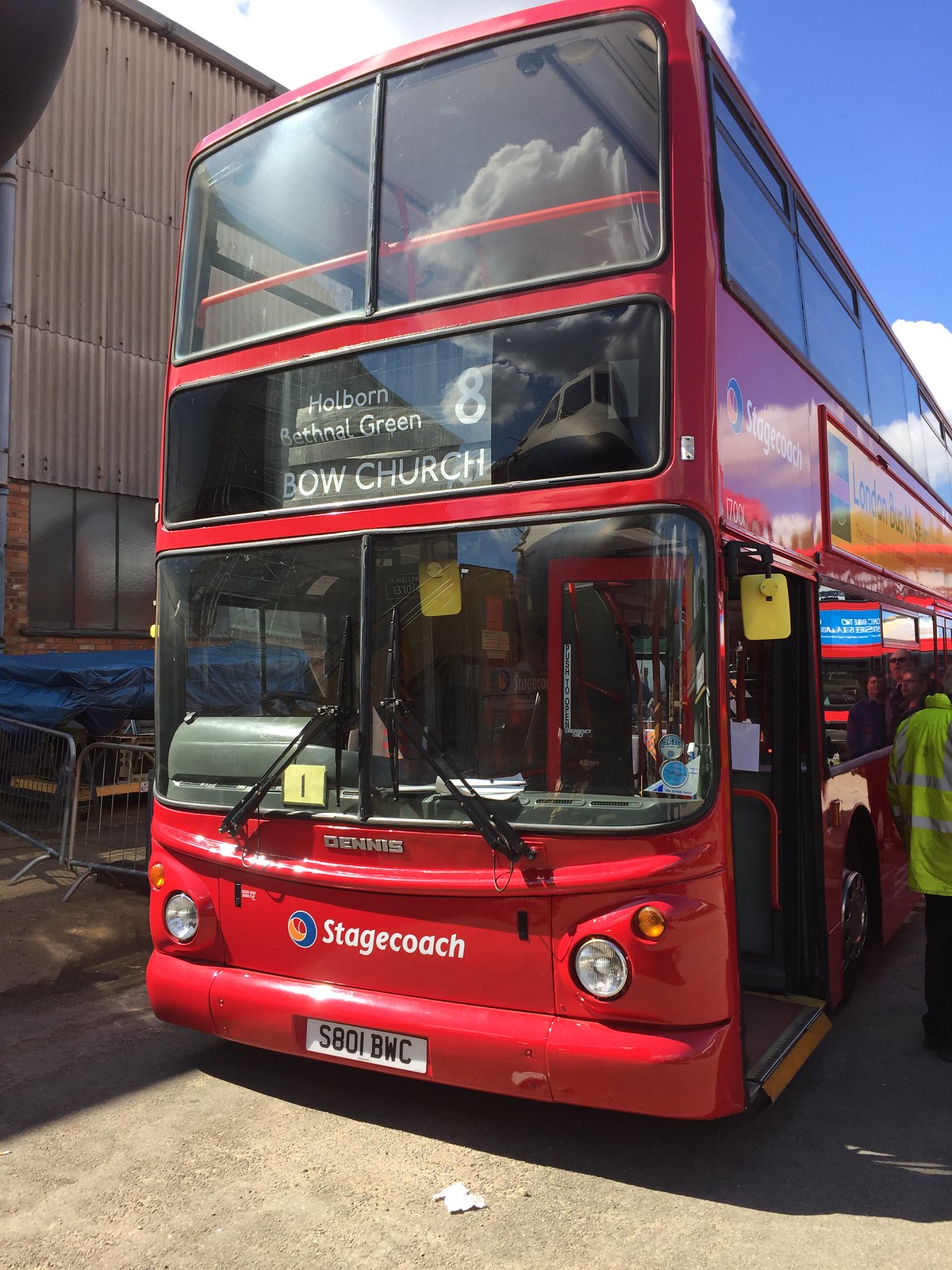This detailed photograph depicts a bright red, modern double-decker bus parked inside a large building that resembles a warehouse. The bus, manufactured by Stagecoach, prominently displays the destination "Holborn, Bethnal Green, 8, Bow Church" on the signage above the driver's window. The license plate reads S801BWC. A distinctive feature of the bus includes its extensive windows that span across the two stories, with additional windows visible on the upper deck. The front of the bus showcases two windows on the top level. Reflections of various advertisements and people can be seen on the side windows. Notably, a person dressed in a yellow high-visibility vest stands near the bus's passenger door, facing away from the camera, though largely cut off and obscured. The scene is captured under sunny, blue skies with white clouds, despite the bus being parked indoors. In the background, a large building with a fenced-in area and a blue tarp is faintly visible through the reflections. The bus appears unoccupied, suggesting it might be stationed for maintenance or inspection.